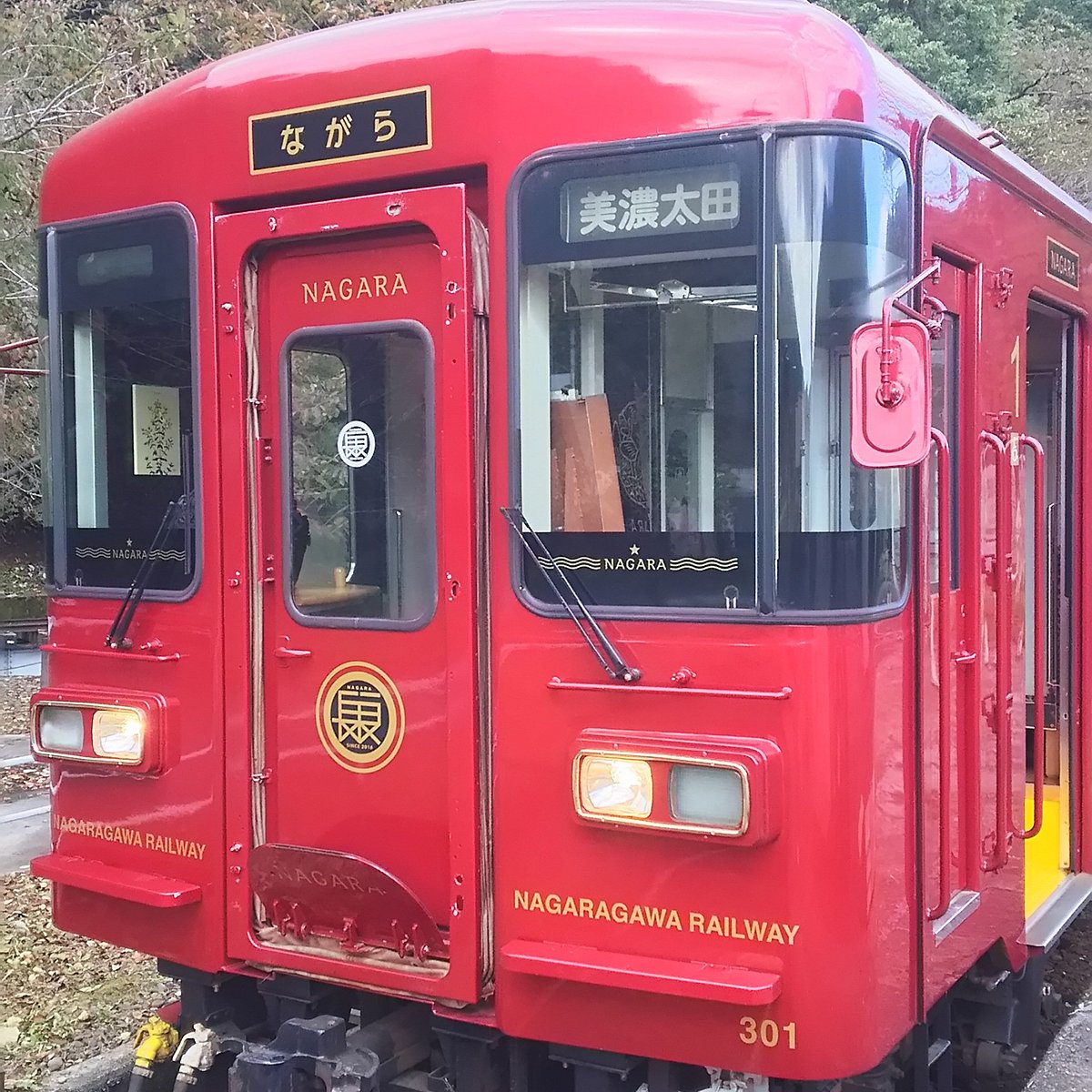The image depicts an outdoor setting featuring a bright red passenger train car, prominently labeled with yellow text. The train car, belonging to the Nagaragawa Railway, displays the word "Nagara" on the front door and the number "301" on the lower right corner. Asian characters, likely Japanese, are visible above the door, adding to the distinctive look. The train car's front also features characteristic elements: black accents above and below the windows, dual windshield wipers resting on two front driver windows, and lights on either side. Machinery and pipes beneath the train hint at its mechanical underpinnings, although the car currently appears idle. The background subtly frames the scene with light green and yellow foliage, hinting at a forested, hilly area, and some visible tracks and roadside elements. The overall impression suggests a well-branded, stationary train in a serene, outdoor environment.